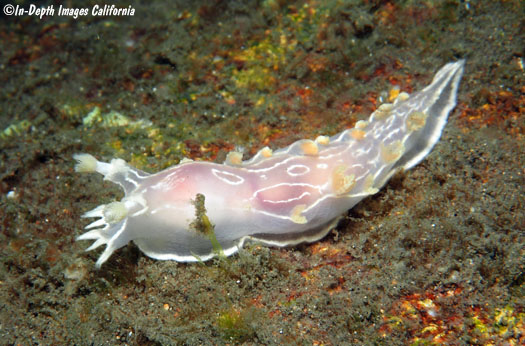This detailed image showcases a captivating sea slug or similar marine creature. Set against an underwater background of granular, sand-like substrate in varying shades of brown, the composition is enriched with patches of bright yellow and dark orange, adding a vibrant contrast. The central subject is a striking white sea slug positioned in the middle of the frame. Its translucent, pale skin reveals underlying hues of darker pink and lighter pink, creating a beautiful and ethereal appearance. The sea slug is further adorned with intricate white circles on its back and tiny raised yellow bumps along its sides, which contribute to its unique texture and natural blending into the mossy, earthy seafloor. The creature's head features small protrusions that resemble eyes, adding to its organic, almost floral appearance. In the top left corner, a copyright symbol reads "In Depth Images, California", anchoring the photo's authenticity.